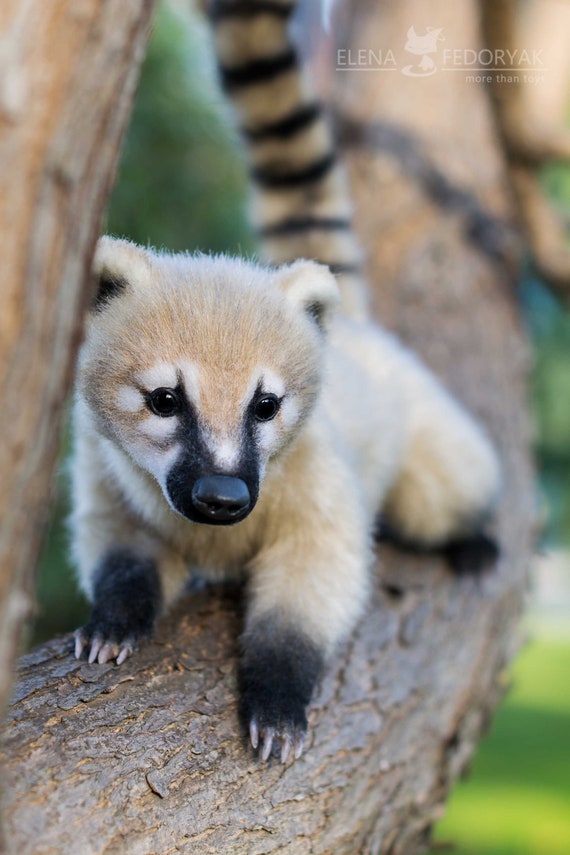The image features an up-close photograph of a small, furry animal that resembles a cross between a miniature bear and a fox, yet also hints at the appearance of a baby badger. It perches on a large, brownish-gray tree branch, clutching with black paws that have four visible claws each. The animal's body is predominantly a pleasing light brown to tan color, accented by darker features. Notable is the black coloration around the nose, extending up to the inside of the eyes, which are wide open, black, and circled with white fur. The ears also have a black portion, but are otherwise brown and small, akin to those of a tiny bear. Adding to its distinctive appearance, the animal sports a long, fluffy tail ringed with black and light brownish-white stripes. The overall look is rounded off with a cute, short fur that covers its petite size. The blurred green background accentuates the detailed subject, and in the upper left corner, there is a watermark with the name "Elena Fedoryak" followed by "Morvan Toys," providing a hint of context about the source of the image.